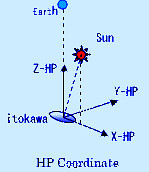The image is a scientific diagram labeled "HP Coordinate" set against a pale blue background with dark blue text and graphics. At its center is an oval from which multiple black lines with arrows extend, each labeled with different coordinates. The line pointing directly upward towards the label "Z-HP" intersects with a dotted line leading to a blue dot labeled "Earth." To the right is an arrow labeled "Y-HP," extending at an upward angle. A dotted line from this arrow leads to a red dot with a black border and beams, labeled "Sun." Another arrow labeled "X-HP" extends downward from the oval. In the lower left of the image, just off-center, is the text "I-T-O-K-A-W-A." This graphic appears to depict an astronomical or geometric relationship, possibly illustrating coordinates or directional vectors in relation to Earth and the Sun.